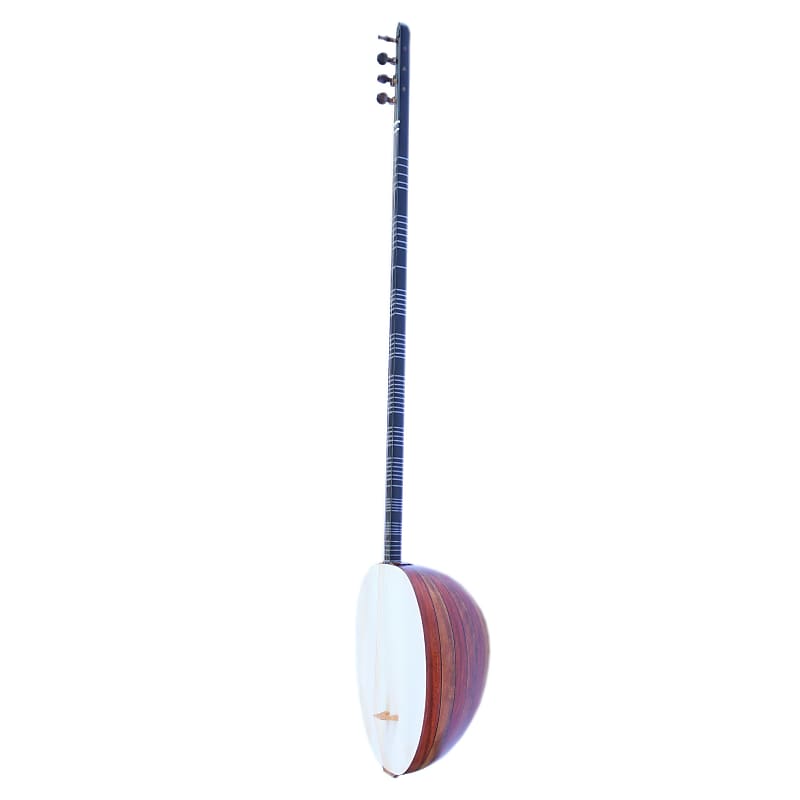This image features a stringed instrument with a unique design, reminiscent of a guitar or banjo but distinctly different. The instrument is positioned vertically against a white background, its details captured from a side profile. The neck, narrower and longer than a traditional guitar's, is a dark blue or black adorned with horizontal white stripes, which might be frets or decorative markings. At the top of the neck, there are four tuning keys, indicating the instrument likely has four strings.

The body of the instrument is shaped like a half-sphere or an oblong oval, with a visually striking combination of red and white tan striped wood around the edges. The front face of the body is a flat, unadorned white, with no visible opening typically found on acoustic instruments. The image is somewhat blurry with blown-out highlights, which obscures finer details but still showcases the instrument's distinctive and elegant construction.